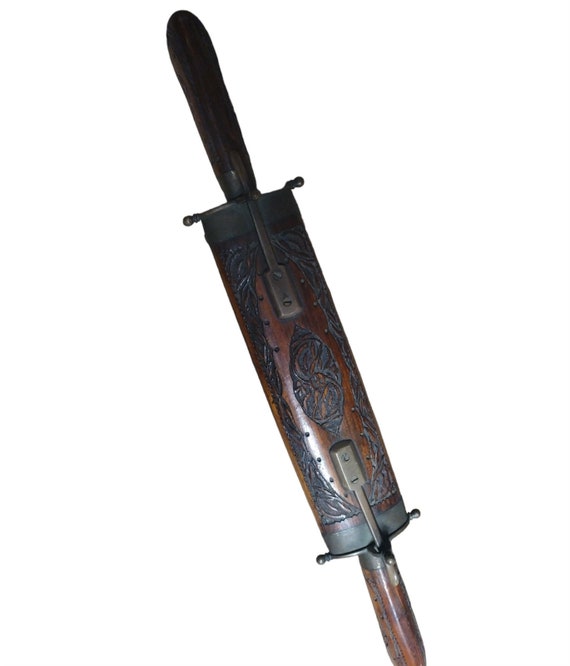The photograph depicts a potentially historic wooden object that resembles a double-sided sheath for swords or daggers, featuring two ornate wooden hilts with T-shaped guards protruding from each end. The sheath is primarily made of dark brown wood and adorned with intricate, abstract carvings and patterns etched into its surface. Metal elements are embedded around the edges and are notably worn, suggesting age. Two metal bars or clasps extend from the top and bottom of the central sheath, connecting to the hilts. The hilts themselves are decorated with ornate designs and have a protective metallic framing at the edges. The background of the image is stark white, highlighting the detailed craftsmanship and aged appearance of the object.